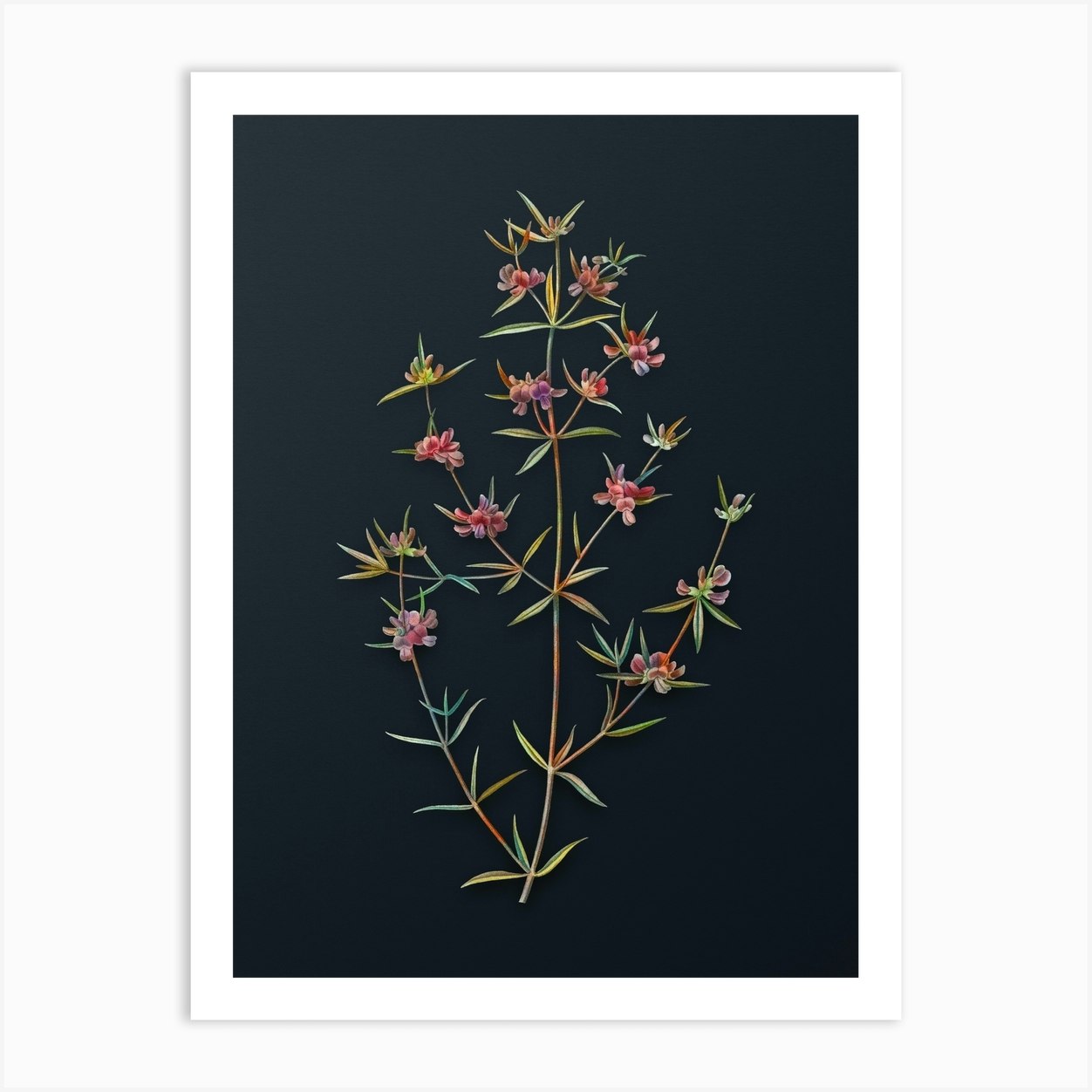The painting depicts a sparse, flowering plant set against a solid black background. The plant has a central stem that branches out into multiple slim, green stems, each adorned with pointy leaves. Some of these stems extend horizontally, while others rise vertically. At the tips and along the sides of these stems, delicate flowers bloom in shades of faint purple, pink, and yellow. Some flowers are fully open, while others are in varying stages of blooming. This vibrant, detailed artwork is mounted in a white frame and displayed on a white wall, with approximately thirteen distinct flowering areas enhancing the plant's airy, graceful appearance.